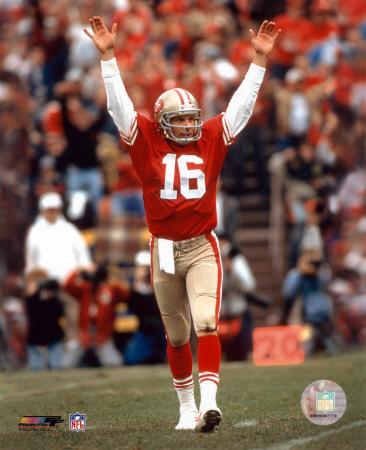This is a detailed photograph of a vintage promotional NFL playing card featuring the legendary quarterback Joe Montana. He is captured on the field, seemingly in a celebratory pose, with both hands raised in the air. Montana is wearing a red jersey prominently displaying the number 16 in white, complemented by a gold helmet with red accents. His uniform includes white long sleeves under the short-sleeved jersey and beige, gold-toned pants adorned with vertical red stripes. His athletic attire is completed with red and white socks and white cleats.

The background of the image shows a slightly out-of-focus crowd seated in the stadium stands, adding to the dynamic atmosphere of the scene. The photograph appears to be taken from a mid-low angle, which gives a powerful perspective, capturing part of the dark green, desaturated turf beneath Montana's feet. 

Adding to the card's authenticity and collector's value, the bottom right corner features a holographic NFL emblem, while the bottom left corner includes another NFL logo and an additional, indistinguishable symbol. A white napkin or towel is also visibly tucked into Montana's pants, enhancing the realism of this iconic football moment.